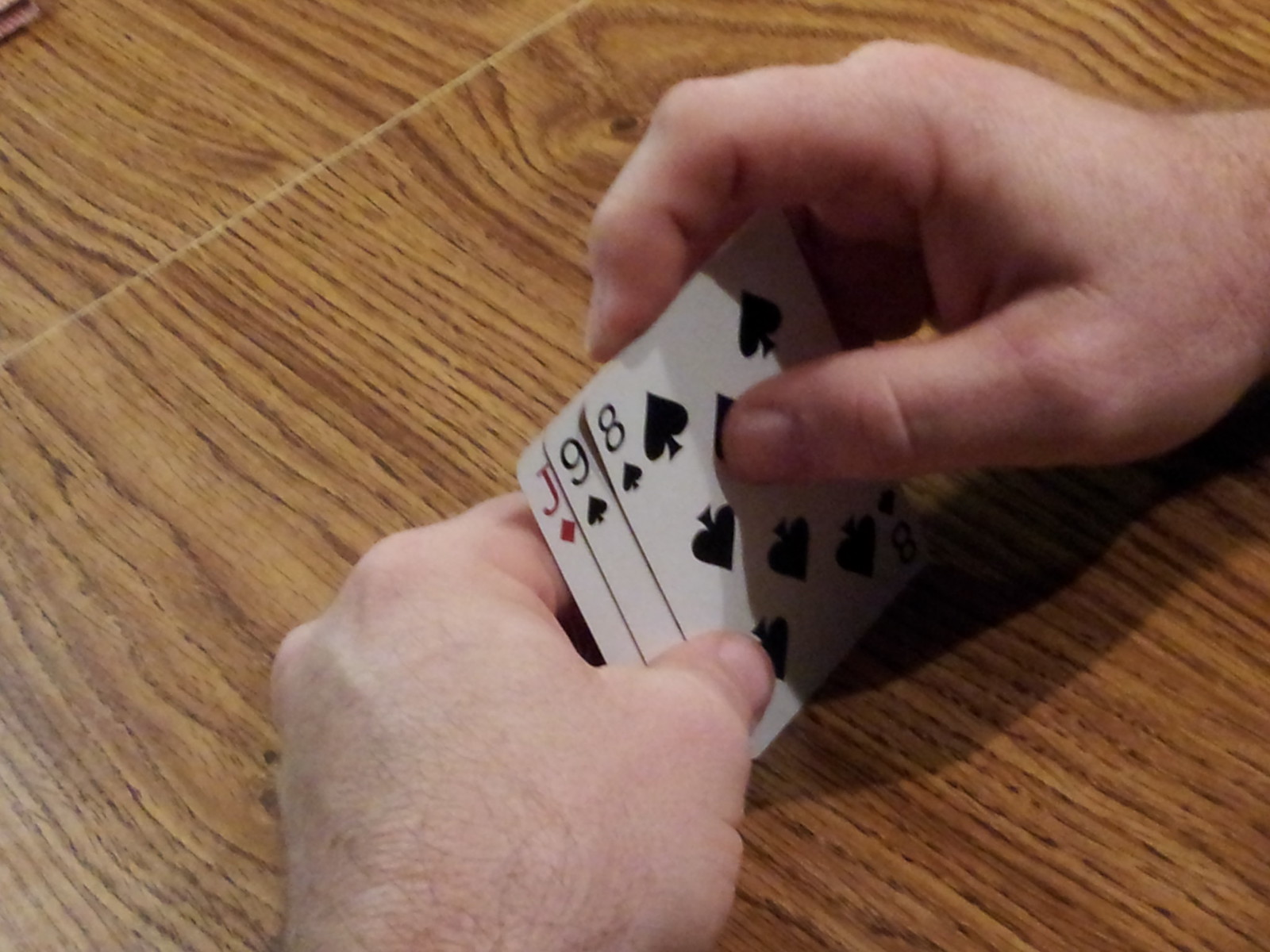In this detailed image, a Caucasian man is depicted holding three playing cards in his left hand while leaning on a light brown tabletop adorned with dark woodgrain lines. He is holding a red Jack of Diamonds, a black Nine of Spades, and a black Eight of Spades, with the cards nestled securely between his left thumb and fingers. His right hand is positioned for a card trick or game, with his thumb pressing down on the far right card and his index finger resting on the top of the cards. A shadow cast by his hand hints at a light source above him. The tabletop features a noticeable horizontal lighter brown line, known as a leaf, and a large circular woodgrain pattern with a darker brown knot above his right hand. The man’s hands and arms are characterized by short, black hair, extending slightly up his arms.